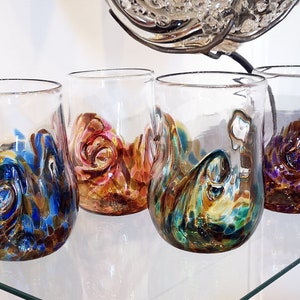This square-shaped image showcases four stemless tumbler glasses arranged on a reflective, shiny white surface. The glasses are adorned with vibrant, abstract designs that cover the bottom two-thirds, with the top third remaining clear. The leftmost glass predominantly features shades of blue, interwoven with subtle variations in color. Next to it, the second glass showcases a striking combination of yellow and red hues. The third glass is a dynamic mix of black, brown, bluish-green, and yellow shades. The rightmost glass primarily displays brown tones with hints of deep purple. Above the glasses, on the right side, a mysterious metallic or glass object extends downward from the top, partially obscured and difficult to identify. The reflections of the glasses on the glossy surface add a compelling depth to the image.